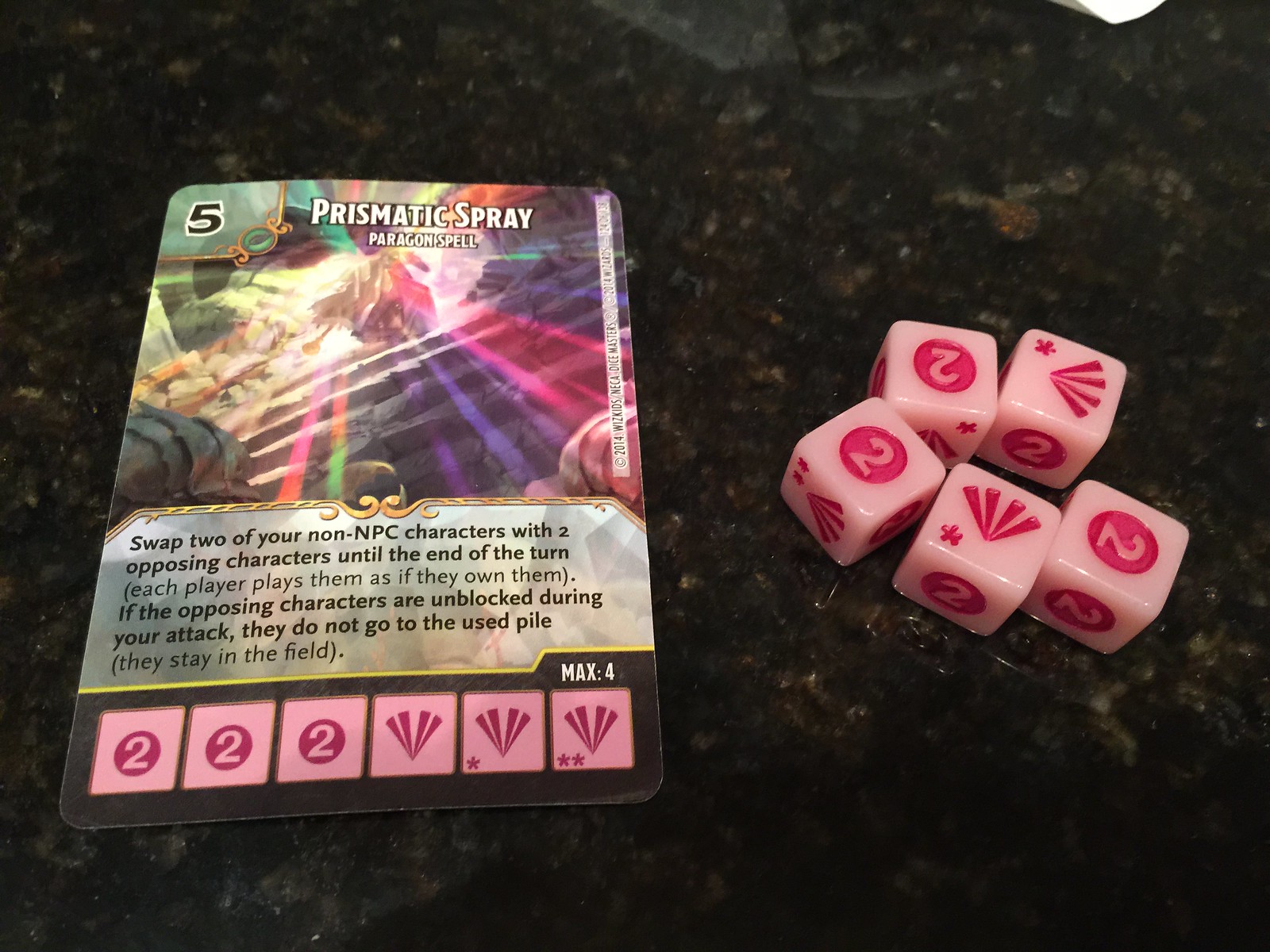In the photograph, a trading card and five dice are set on a sleek, black marble countertop, interspersed with various colored field stones. The card, oriented vertically on the left, features a complex, colorful image resembling rays of light in shades of purple, magenta, green, and red. At the top left of the card, a black number "5" with a white border is visible. Directly to the right, white text on a black-bordered strip reads, "Prismatic Spray, Paragon Spell." Below this, in a gray box with black text, are the instructions: "Swap two of your non-NPC characters with two opposing characters until the end of the turn. Each player plays them as if they own them. If the opposing characters are unblocked during your attack, they do not go to the used pile. They stay in the field."

The bottom section of the card showcases a series of six pink squares. The first three squares each contain a white number "2" within a pink circle. The last three squares feature a fan-shaped diagram with varying star details: one with no star, one with a star in the top left corner, and the last with two stars in the bottom left corner.

To the right of the card lie five dice. Two dice display the fan-shaped symbol with stars, and the remaining three dice show the number "2" within a pink circle, mirroring the card’s bottom sequence. This meticulously detailed setup highlights the intricacies of the card's gameplay function and design, all presented on an elegant marble surface.